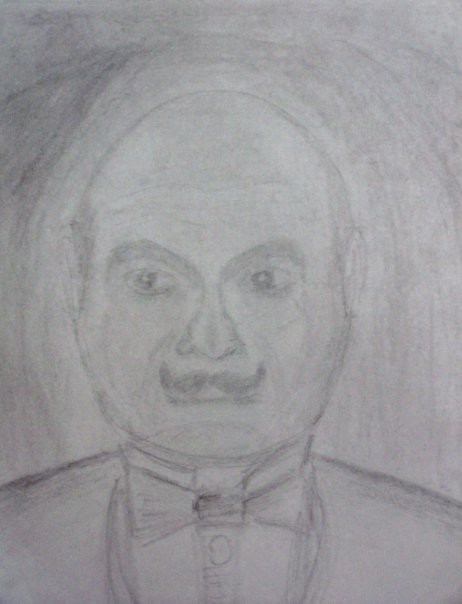A highly detailed pencil drawing depicts a balding man with a distinctive look, characterized by hair only on the sides of his head similar to a monk's tonsure. He wears a suit jacket with narrow lapels, a bow tie shaped like a candy wrapper with a central cylinder, and a visible shirt button. The man has expressive, arched eyebrows, dark eyes with white dots in the pupils, a broad nose, and a prominent mustache reminiscent of Hercule Poirot's. His face, marked by subtle shading to suggest wrinkles on his forehead, conveys age and experience. He gazes slightly to his right, though the object of his attention is not visible. The entire piece, rendered solely in pencil, demonstrates significant artistic skill, particularly through the detailed shading that enhances the depth and texture of the portrait. The background features extensive shading, which accentuates the finely drawn subject, emphasizing the skill of the artist.